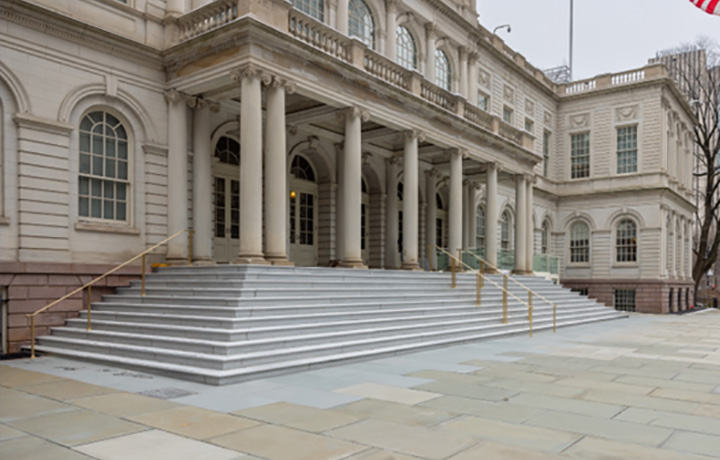This photograph captures the detailed exterior of an old-fashioned, two-story building constructed from light tan, antique-looking marble and granite blocks used for the foundation. The structure features a series of wide, granite steps, approximately 15 in total, that lead up to a grand entrance. The steps curve around to the side, with brass railings to assist those ascending or descending. There are sets of columns arranged in a distinctive formation: double pillars on either end and four pillars in the middle, supporting a portico or upper balcony area. The balcony, also made of stone, features intricate stone railings and overlooks the steps below. The building's many windows are prominent, particularly the arched windows with rectangular bases that contribute to the building’s textured and historic appearance. Additionally, a small piece of a flag can be seen waving in the upper right corner, adding a touch of color to the scene. The overall look of the building, with its numerous pedestals and coliseum-like resemblance, exudes a classical, timeless elegance.